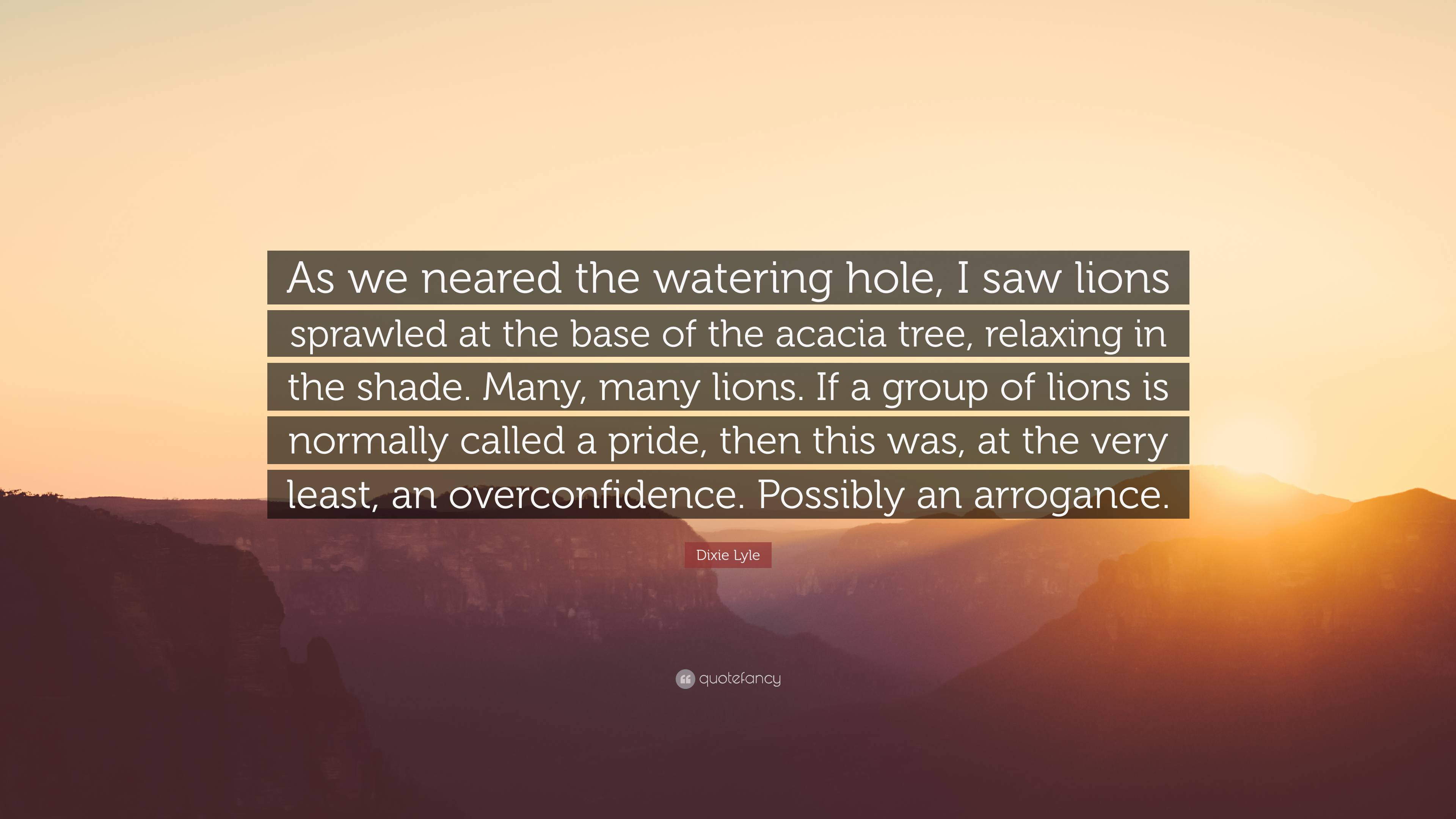The image features a serene landscape of expansive mountains bathed in the soft, peach-hued light of either a setting or rising sun. The sky's gradient ranges from light orange to pink, contrasting subtly against the silhouetted mountains. At the heart of the image, a series of gray rectangular bars are overlaid, carrying a poignant quote in white text: "As we neared the watering hole, I saw lions sprawled at the base of the acacia tree, relaxing in the shade. Many, many lions. If a group of lions is normally called a pride, then this was, at the very least, an overconfidence, possibly an arrogance." The quote is attributed to Dixie Lyle, noted within a reddish box with white text at the bottom. The overall aesthetic is enhanced by the serene background, with the text presented in a typewriter-style serif font, adding a classic touch to the depicted scene.